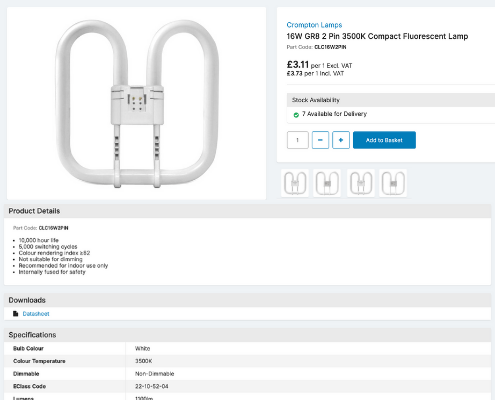A detailed image depicting a webpage product listing for a Crampton Lights compact fluorescent lamp. The screenshot has a light gray border and white background, with various sections and text descriptions as follows:

* **Top Left Corner:** An image of a fluorescent light bulb with squared curved edges, converging at the top into a square area where the bulb hooks into the fixture. Two vertical connections extend downwards, meeting the bulb tube at the base.

* **Text to the Right of the Image:** 
  * In blue lettering, "Crampton Lights" (capitalized C and L).
  * Below in black lettering: "16W GRB, 2 PIN, 3500K Compact Fluorescent Lamp" (with capitalized letters as indicated).

* **Additional Details Beneath the Text:**
  * In gray lettering, a part number, partially obscured, followed by a price listed in black: "£3.11" with smaller, lighter text detailing the price.
  * Availability indicated by a green circle stating "2 Available for Delivery" in black lettering.

* **Interactive Elements:**
  * A gray bar with "Stock Availability" (capitalized S and A).
  * Below the availability note, control boxes: 
    * A gray box with the number "1".
    * A blue box with a minus sign.
    * A blue-border box containing a plus sign, both symbols in blue.

* **Action Button:** A blue rectangular button with white text reading "Add to Basket" (capitalized A and B).

* **Product Details Section:**
  * A gray bar with "Product Details" (capital P and D).
  * Below, in light gray lettering, a part code or number accompanied by black letters/numbers, partially obscured and blurry.
  * A series of six bullet points, each with a corresponding explanation.

* **Downloads Section:**
  * A gray bar with "Downloads" (capital D), with a white background beneath featuring a black box and blue text initially appearing to spell "D" (indicative of a downloadable link).

* **Specifications Section:**
  * Another gray bar with "Specifications" (capital S).
  * Below, five rectangular boxes with alternating background colors (white and gray), featuring black text:
    * The first specification line reads "Color: White" (with relevant capitalization and vertical line separator).
  * Further specifications are listed with a repeating background color scheme, including a class code "22-10-52-04" and a partly obscured final text.

This detailed description captures all significant elements and text visible within the screenshot, providing a comprehensive overview of the product listing.